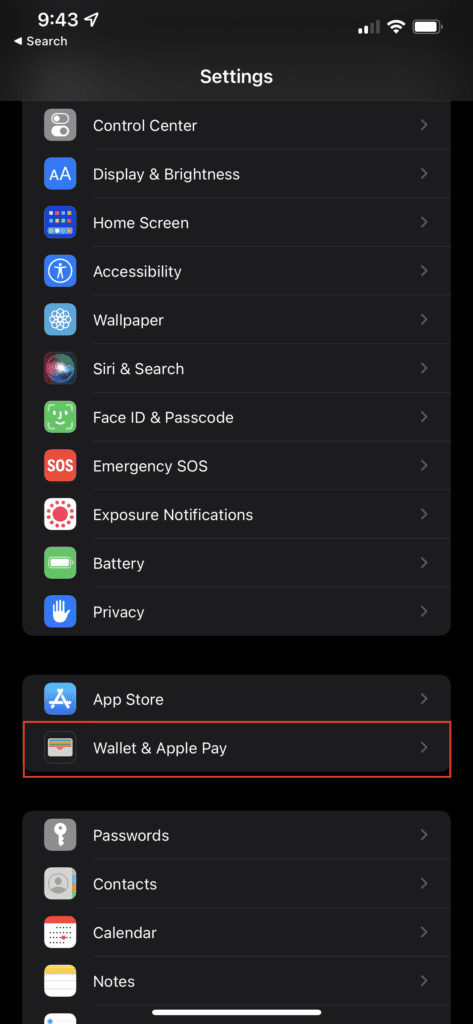The image depicts a black screen with various elements and text. At the top, it displays the time as 9:43, along with an arrow symbol, indicating a navigation option. The status bar shows 2 out of 4 bars of signal strength, Wi-Fi connectivity, and battery life. Below this, a list of settings options is visible, including:

- Search
- Settings
- Control Center
- Display & Brightness
- Home Screen
- Accessibility
- Wallpaper
- Siri & Search
- Face ID & Passcode
- Emergency SOS
- Exposure Notifications
- Battery
- Privacy
- App Store
- Wallet & Apple Pay
- Passwords
- Contacts
- Calendar
- Notes

A white bar is located at the bottom of the screen, likely representing a gesture bar. The "Wallet & Apple Pay" option is highlighted with a red square around it, drawing attention to this particular setting.